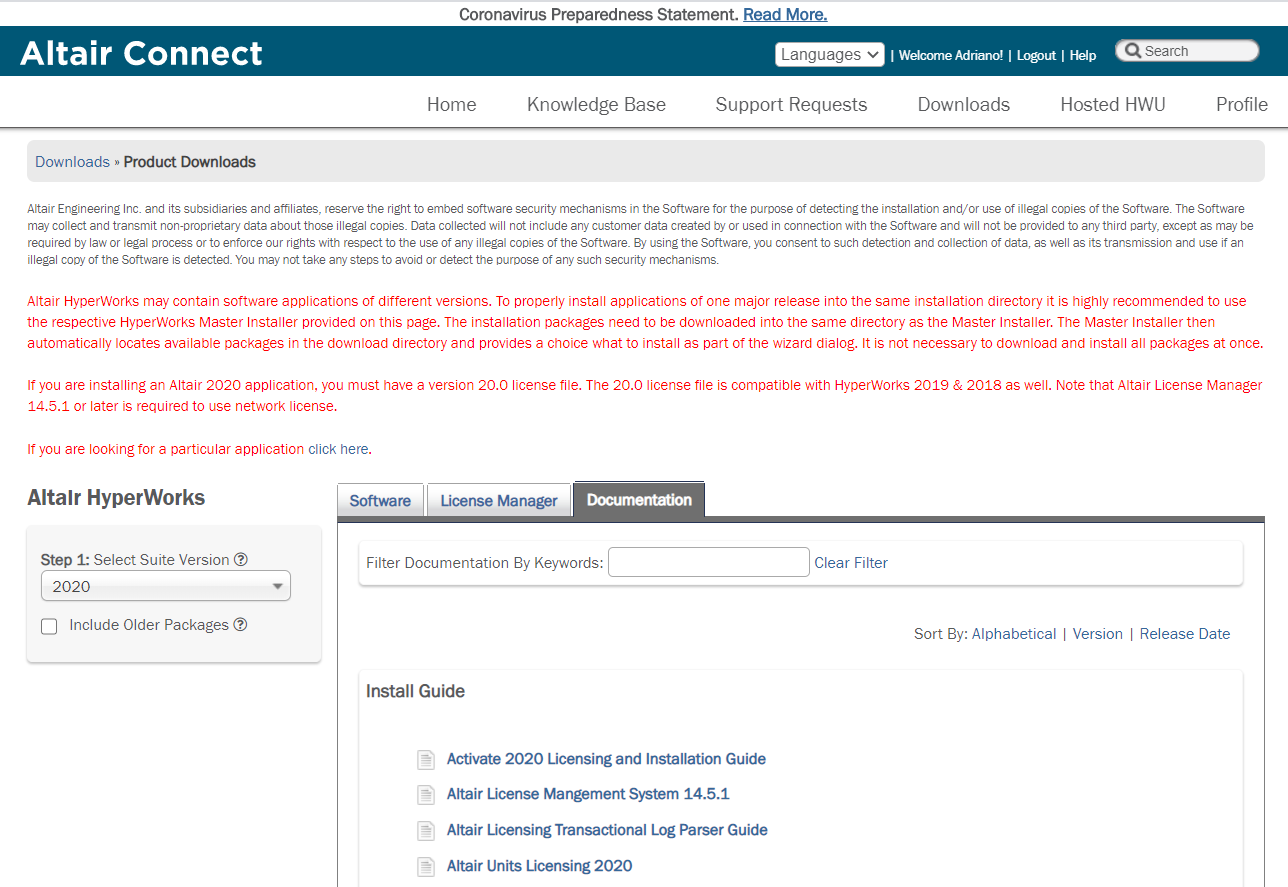**Detailed Caption for a Coronavirus Preparedness Statement Document:**

The image captures a coronavirus preparedness statement document, designed for users accessing the ALT AIR Connect system. The document is structured on a white background and features a prominently displayed blue header at the top. The header, in bold white letters, reads "ALT AIR Connect." Adjacent to this title, there's a languages dropdown menu, offering various language options. Just to the right of this menu, the page greets the user with the text, "Welcome Adriano!" followed by an exclamation mark.

Further to the right within the header, there are quick-access buttons including "Logout," "Help," and a "Search" function icon. Below the header, a series of hyperlinks provide easy navigation to different sections: "Homepage," "Knowledge Base," "Support Requests," "Downloads," "Exit HWU," and "Profile."

Under its dedicated "Downloads" section, the document stresses the importance of software security by ALT AIR Engineering Incorporated. It mentions ALT AIR's right to embed security mechanisms in its software to detect and prevent the use of illegal copies. Detailed information is provided regarding the data collection process, ensuring users that no customer data will be included or shared with third parties, except under legal obligation. Consent is implicit upon using the software, and attempts to circumvent these security protocols are prohibited.

The document further details the installation instructions for ALT AIR HyperWorks applications, indicating the necessity of a master installer for a seamless setup of multiple software versions within the same directory. Specific instructions for installing the 2020 version of ALT AIR applications call for a 20.0 license file, noting its compatibility with previous versions from 2019 and 2018. Additionally, it emphasizes the need for ALT AIR License Manager 14.5.1 or later for network license use.

An instructional section outlines how to navigate software version selection with a highlighted "Step 1 Select Suite Version" box, which currently displays "Version 2020." There is an option to include older software packages. At the bottom right of the document, three essential links are provided for further actions: "Software," "License Manager," and "Documentation." The current view is on the "Documentation" link, which includes a keyword filter for easy documentation search, coupled with sorting options such as "Alphabetical," "Version," and "Release Date."

Finally, at the very bottom, an installation guide section is displayed, offering four specific links for users:
1. "Activate 2020 Licensing and Installation Guide"
2. "ALT AIR License Management System 14.5.1"
3. "ALT AIR Licensing Transactional Log Parser Guide"
4. "ALT AIR Units Licensing 2020"

This detailed structure ensures users can navigate and understand the document comprehensively, bolstering their preparedness and compliance with ALT AIR's software guidelines amidst COVID-19 concerns.